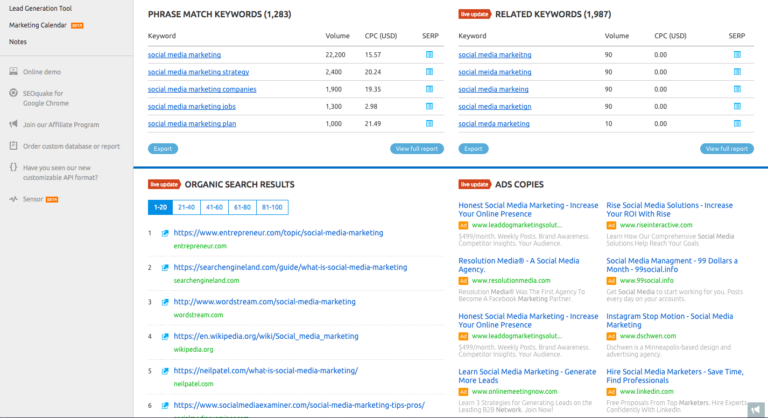This image is a screenshot of a page detailing various features related to a lead generation tool. At the top of the page, the title "Lead Generation Tool" is prominently displayed. Below it, there's a "Marketing Calendar" section labeled "Beta" with an orange tag. 

To the right, a "Notes" section is visible alongside options such as "Online Demo," "SEOquake for Google Chrome," "Join our Affiliate Program," and "Order Custom Database or Report." Additionally, there's a mention of a new customizable API format and a "Sensor" feature, also tagged as "Beta."

In the center of the screen, there's a highlighted section labeled "Phrase Match Keywords" listing a total of 1,283 keywords. Some of the keywords include "social media marketing," "social media marketing strategy," "social media marketing companies," "social media marketing jobs," and "social marketing plan." Each keyword is accompanied by metrics such as volume, CPC (Cost Per Click) denoted in USD (USD), and SERP (Search Engine Results Pages) position.

Adjacent to this is a "Related Keywords" section listing 1,987 related keywords, with a highlighted keyword "social media marketing" showing a volume of 90 and SERP data.

At the bottom of the page, there’s an "Organic Search Results" section displaying a variety of links ranked in increments of 1-20, 21-40, 41-60, 61-80, and 81-100. Additionally, an "Ads Copies" section shows different clickable ad links.